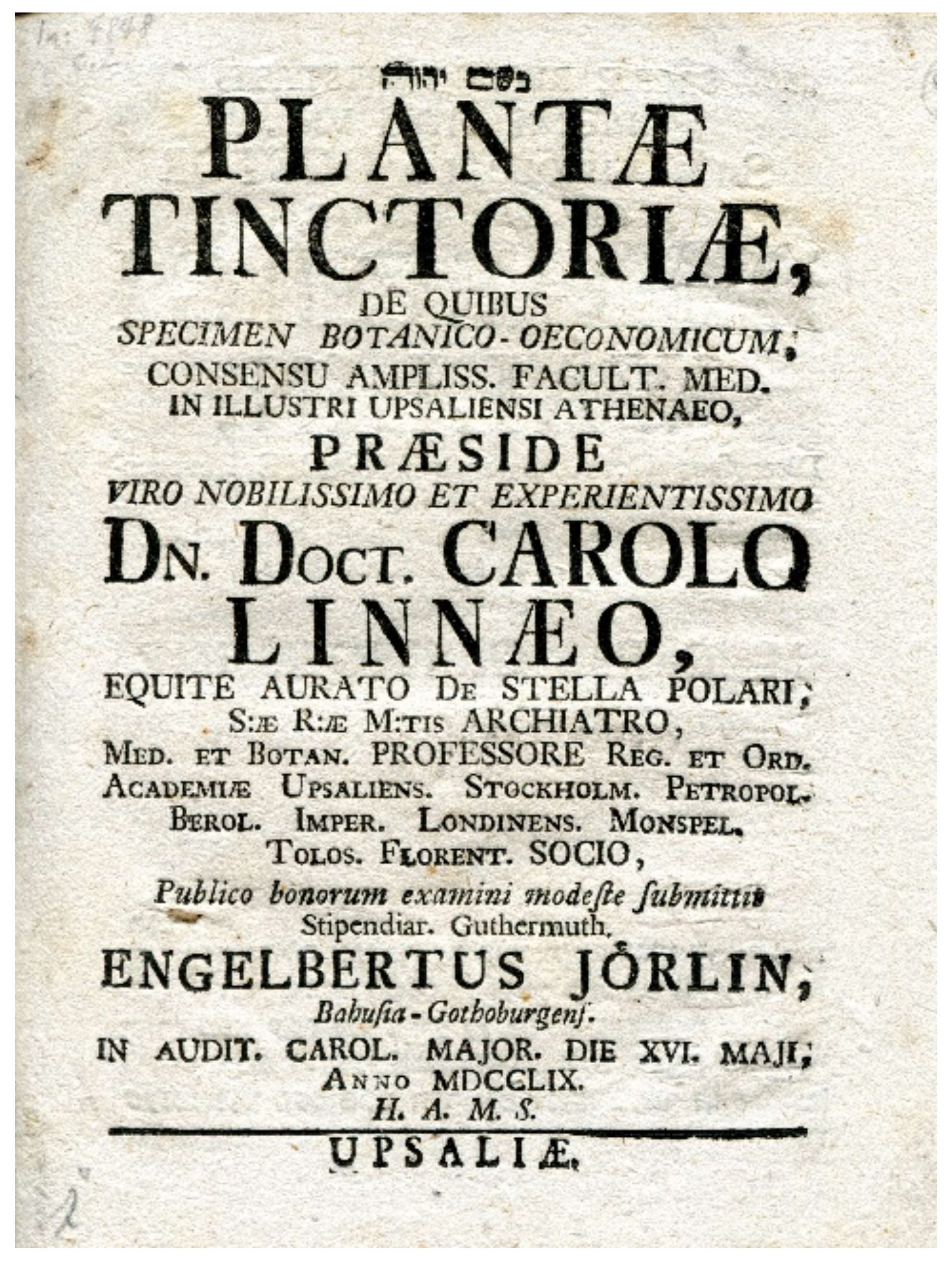The image depicts an old paper or flyer, resembling a historical document, written in Latin. The page features black lettering on a whitish-gray mottled background and includes various fonts throughout. At the top, there's a prominent headline that reads "Plantae Tinctoriae." Below that, in smaller text, appears a Latin description that includes phrases such as "decibis, specimen botanico, oceanum, consensu amplis, faco med, in illustri, unspellensi, atianzo." Mentioned on the page are terms that seem to relate to botanical or medical subjects, possibly discussing the treatment or impact of a certain plant. Notable names and locations such as "Stockholm" and "Jorlan Engelbertus" are also present. Furthermore, there's a presentation to "dn.doct.carlolaneo," suggesting the document could be a form of award or recognition. The overall appearance is reminiscent of a flyer that one might see stapled to a telephone pole to announce or advertise something.